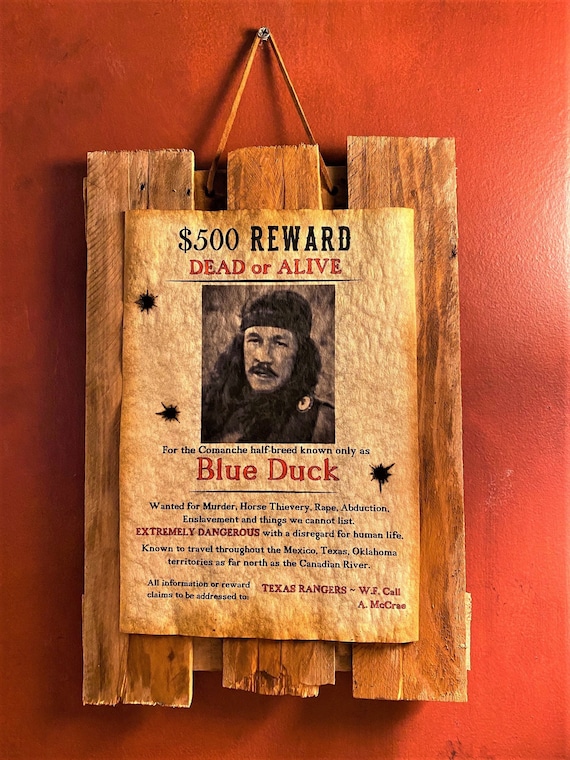The image features a vintage-styled, computer-generated poster designed to replicate an old wanted notice. It is affixed to a wooden plaque, composed of three vertically aligned boards, hanging on a nail against a textured, dark burnt-red wall. The worn paper on the plaque, with crisp burnt or dirty edges tinged brown, prominently displays a "WANTED: DEAD OR ALIVE" notice, offering a $500 reward. The heading "REWARD" is highlighted in bold, black uppercase letters, while "DEAD OR ALIVE" is also bolded for emphasis.

Central to the poster is an illustration of the fugitive known as Blue Duck, a Comanche half-breed characterized by his tied-back hair adorned with a headband and a fur-trimmed garment around his neck, giving a neutral expression. The name "BLUE DUCK" is the largest text after "REWARD," signifying his notoriety. The poster declares Blue Duck wanted for severe crimes, including murder, horse thievery, rape, abduction, enslavement, and unspecified heinous acts. His extreme danger and lack of regard for human life are noted in red uppercase font.

The poster further mentions that Blue Duck operates across the Mexico, Texas, and Oklahoma territories, reaching as far north as the Canadian River. All information or reward claims are directed to the Texas Rangers, under the names W.F. Call and A. McRae. The poster is stylistically marked by three bullet holes, adding to its aged and gritty aesthetic.